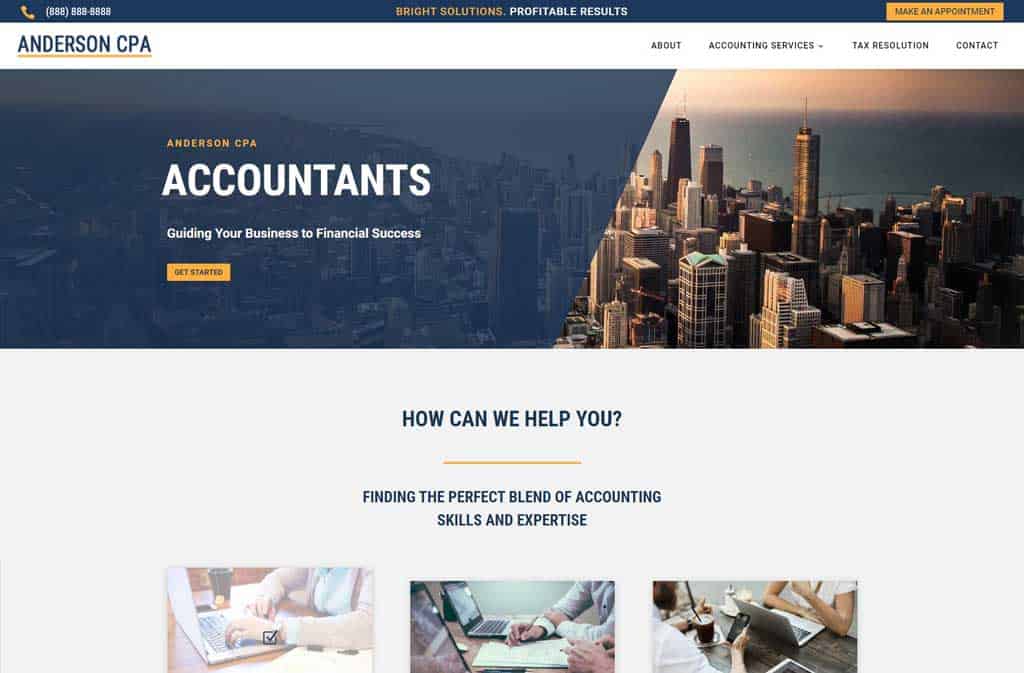**Website Banner Description for Anderson CPA:**

At the very top of the website, a sleek navy blue banner prominently features key contact information and company branding. On the left, a phone icon is followed by the company’s contact number: (888) 888-888. Centrally located in this banner, the company’s tagline "Bright Solutions" is elegantly highlighted in gold, paired with "Profitable Results" in crisp white text, providing a strong first impression. To the right, a bold gold rectangle catches the eye with the call-to-action "Make an appointment" in navy blue. 

On the left, the company name "Anderson CPA" stands out in navy blue text, underlined by a refined gold line for emphasis. Navigation options follow to the right, featuring categories such as "About," "Accounting Services," "Tax Resolution," and "Contact."

Dominating the background is a beautifully rendered cityscape of a large metropolitan area, adding a touch of modernity and scale. Partially overlaying this cityscape with a block of blue-gray color, "Anderson CPA" is repeated in striking gold text. Below it, "Accountants" appears in really large bold letters, complemented by the tagline "Guiding Your Business to Financial Success" to reinforce the firm’s commitment to client prosperity.

Towards the lower section, another gold rectangle draws attention with a "Get Started" button, inviting user engagement. Below, the text "How can we help you?" in gray is followed by a gold line and the phrase "Finding the perfect blend of accounting skills and expertise," which encapsulates the firm’s dedication to exceptional service.

This detailed webpage design artfully combines important visual and textual elements to present Anderson CPA as a professional, approachable, and results-driven accounting firm.